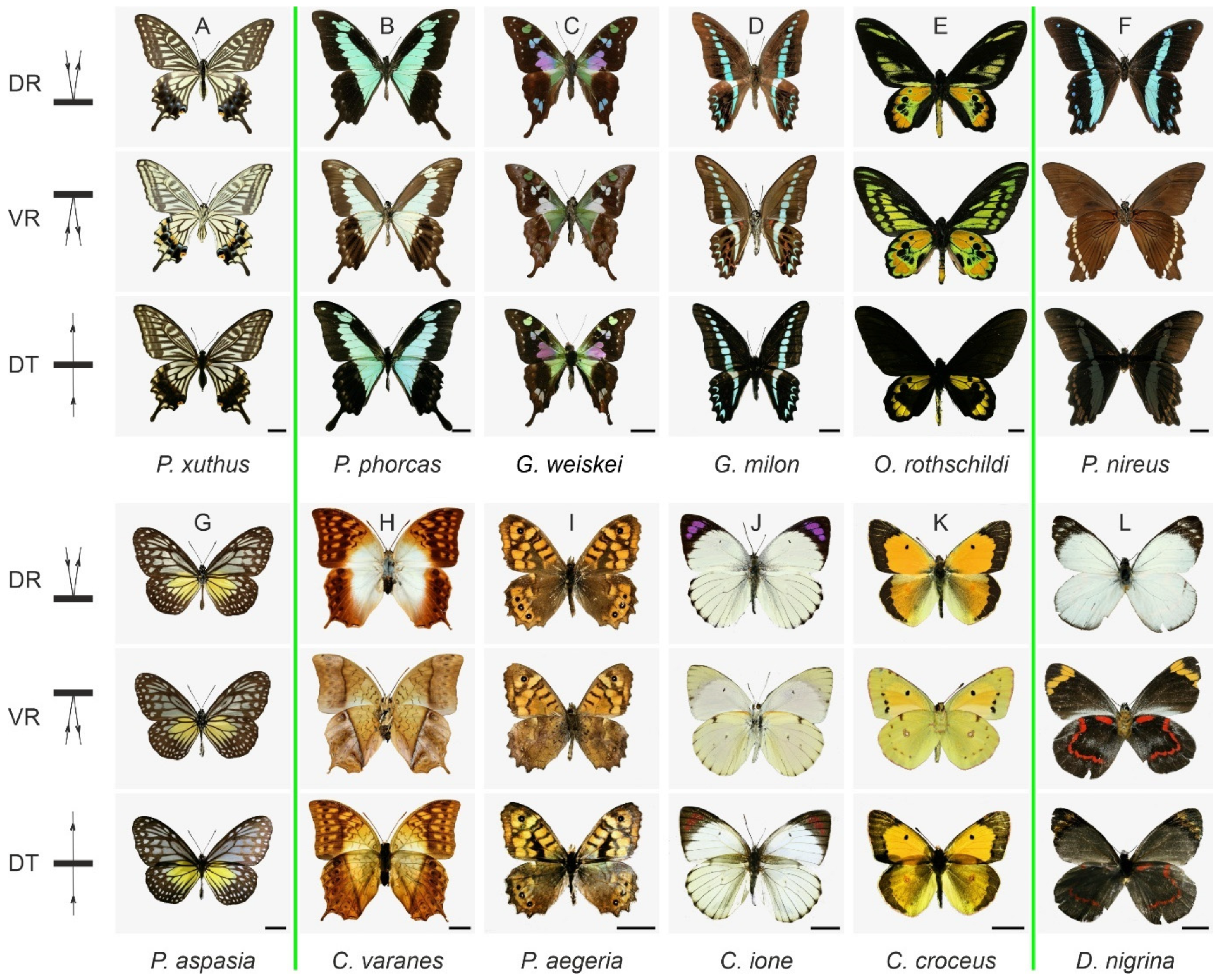The image is a detailed scientific classification chart of various butterfly species, organized in a large vertical rectangle with a white background. The butterflies are arranged in horizontal rows of six, with three sections containing two rows each, for a total of six rows. Each row is systematically labeled both horizontally and vertically. 

At the top, columns are designated by letters A through F. On the left side, labels run vertically in a repeating pattern of "DR", "VR", "DT", "DR", "VR", "DT" from top to bottom. The butterflies in the top half are sharper and more pointy, while those in the lower half are rounded.

In the center of the chart, specific butterfly species are labeled sequentially across the rows: 
- Top rows (grouped together): P. xuthus, P. phorcus, G. weiskei, G. millen, O. rothschildi, and P. nireus.
- Bottom rows: P. aspasia, C. varengs, P. aegeria, C. ione, C. croceus, and D. negrina.

Notably, a lime green line separates the columns on the far right and the far left from the rest of the chart, adding a distinct visual element to the classification layout.